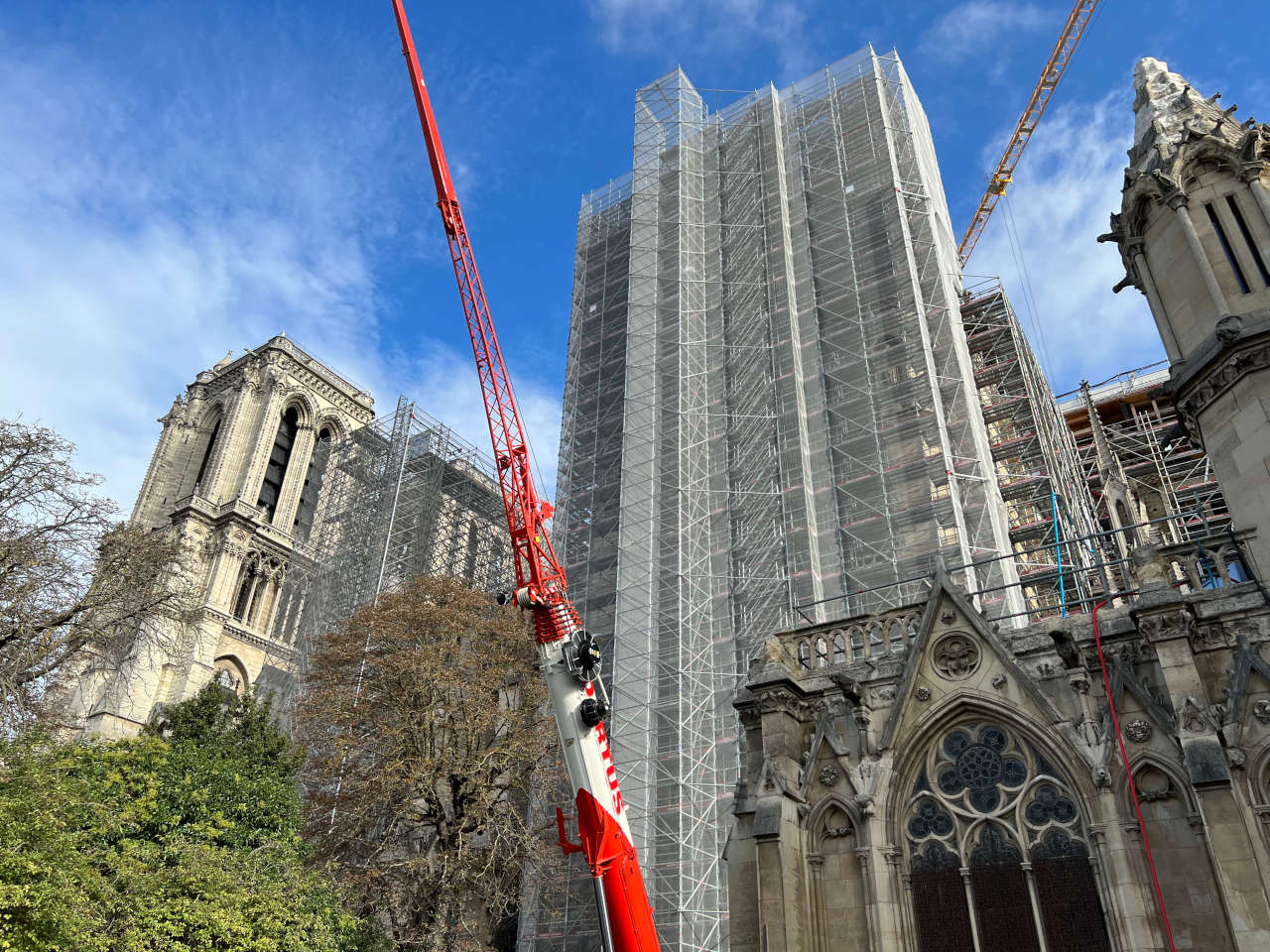This daytime photo captures a Gothic-style cathedral undergoing renovation. The image, taken from a ground perspective looking upward, prominently features scaffolding surrounding a tower to the left side of the cathedral, indicating active construction work. The cathedral, made of gray stone with intricate designs, has blacked-out window spaces and an untouched section on the right that showcases its original architectural elements, including an arched door and pointed tower. Several cranes are visible, particularly one orange crane in the center and a white and red crane on the left, which has "RTUS" marked on it. Additionally, a white and red pipe can be seen to the right of the building under renovation. The sky above is blue with white clouds, and greenery, including trees and bushes, is present at the bottom left corner and along the bottom of the image, suggesting a garden space adjacent to the cathedral.